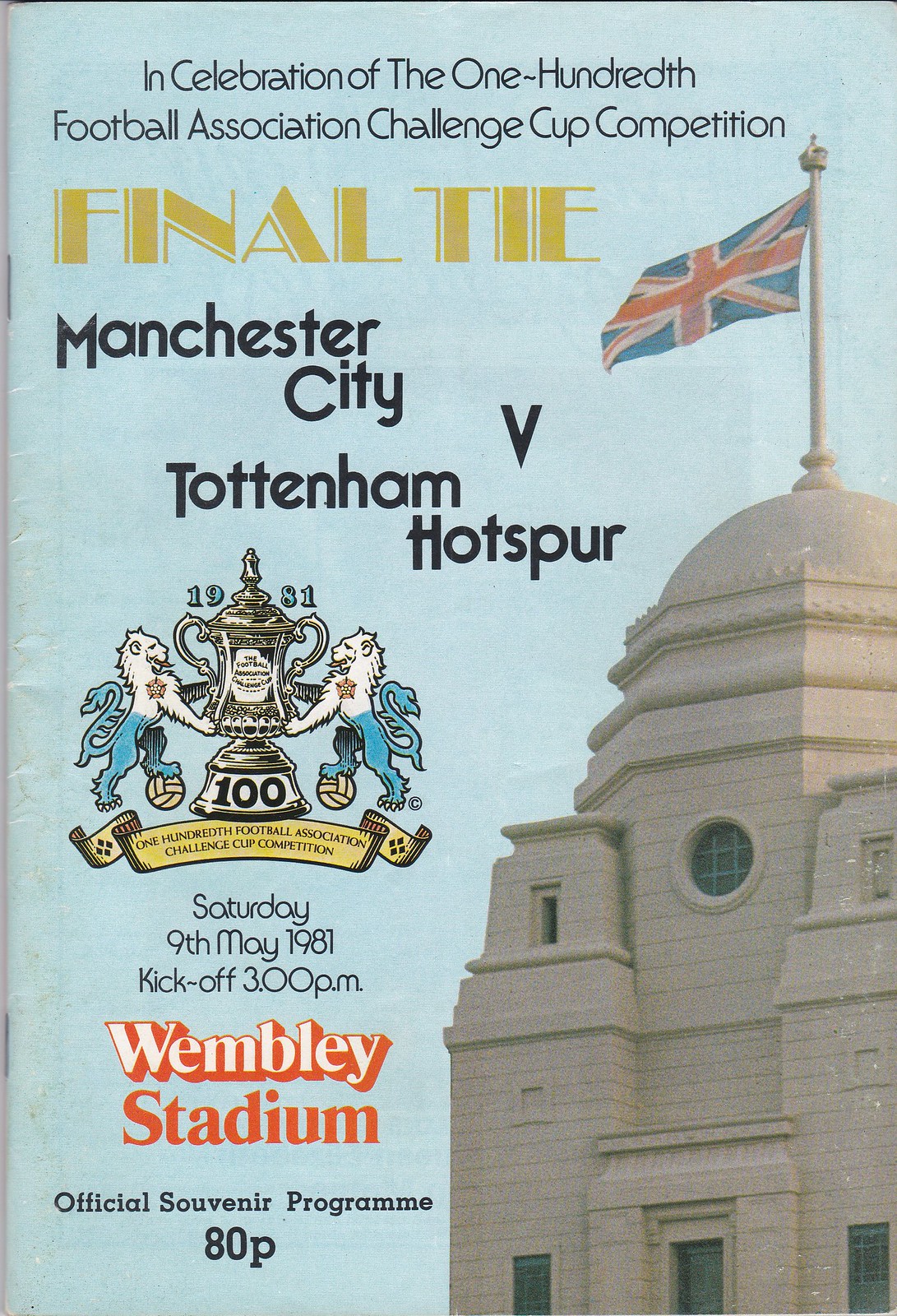The cover of the official souvenir program for the 100th Football Association Challenge Cup Competition features a vertically aligned rectangular image with two staples on the left where the spine is, accompanied by visible wrinkles along the spine. The background showcases a light blue sky with textual content overlaid in this area. At the top, black text reads, "In celebration of the 100th Football Association Challenge Cup Competition." Below this, in large, gold, all-caps letters, it says, "FINAL TIE." Further down, in bold black text, it lists, "Manchester City vs. Tottenham Hotspur." There is an illustration beneath this text, depicting two creatures with curled tails and a blue lower half, holding a silver and gold trophy labeled "100." Above the trophy, the year "1981" is prominently displayed. Under this image, in small black text, it specifies, "Saturday, 9th May 1981, kickoff 3 p.m." The text "Wembley Stadium" is prominently placed below in white and red text respectively. The bottom left corner bears the small inscription, "Official Souvenir Program ADP." The right side of the cover is dominated by a stone building with a dome top, from which a British flag is flying, adding a sense of grandeur and historic significance to the program.